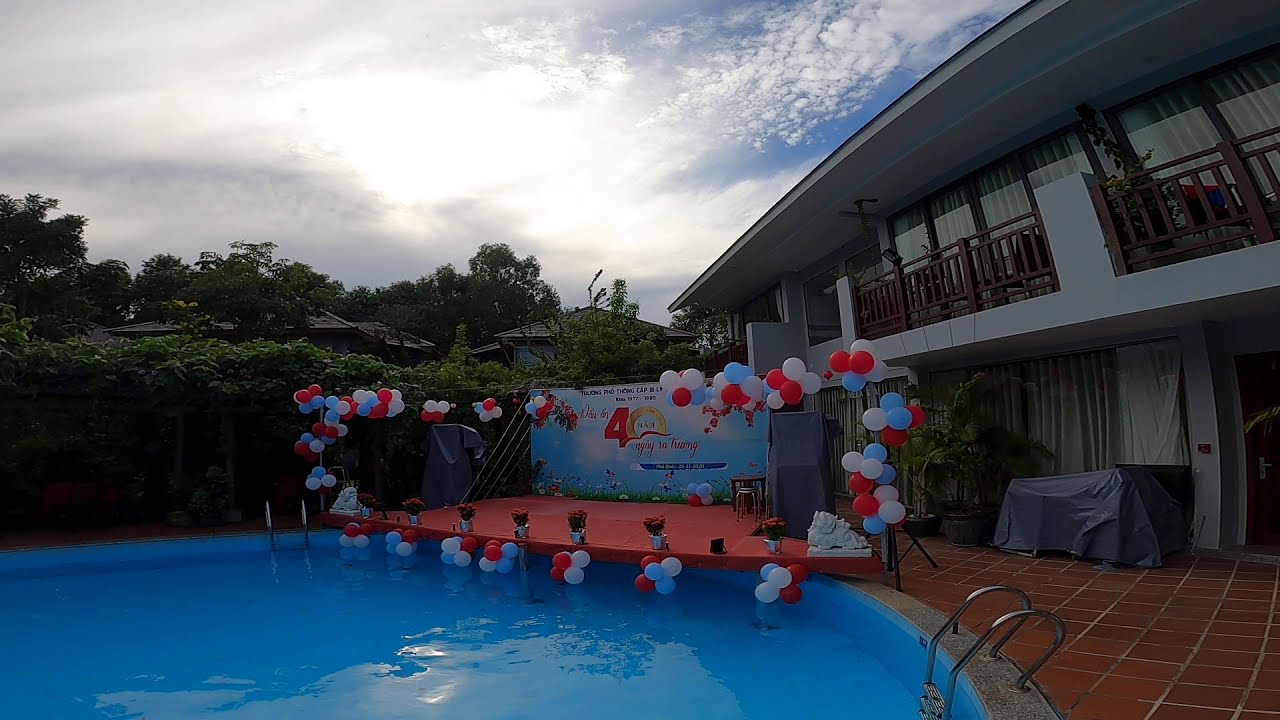The image depicts an outdoor party scene at a two-story hotel with a red brick patio and numerous windows adorned with red wrought iron railings and balconies. Dominating the foreground is a rounded pool with clear, aqua-colored water, likely from blue tiled flooring. Adjacent to the pool is a vibrant red stage festooned with red, white, and blue balloons, celebrating an event marked by a prominently displayed "40," though the exact occasion is indecipherable due to the foreign text, possibly Japanese. Beyond the stage, there are lush green bushes and trees interspersed with housetop glimpses. The sky overhead is clear blue with scattered white clouds. On the right side of the image, near the pool, a table is visible along with tall structures cloaked in black tarps. Covering the scene, the upper level of the building features large curtained windows or sliding doors, while the lower level includes additional covered areas and large potted plants. The setting appears tropical, suggesting a festive, yet tranquil atmosphere.